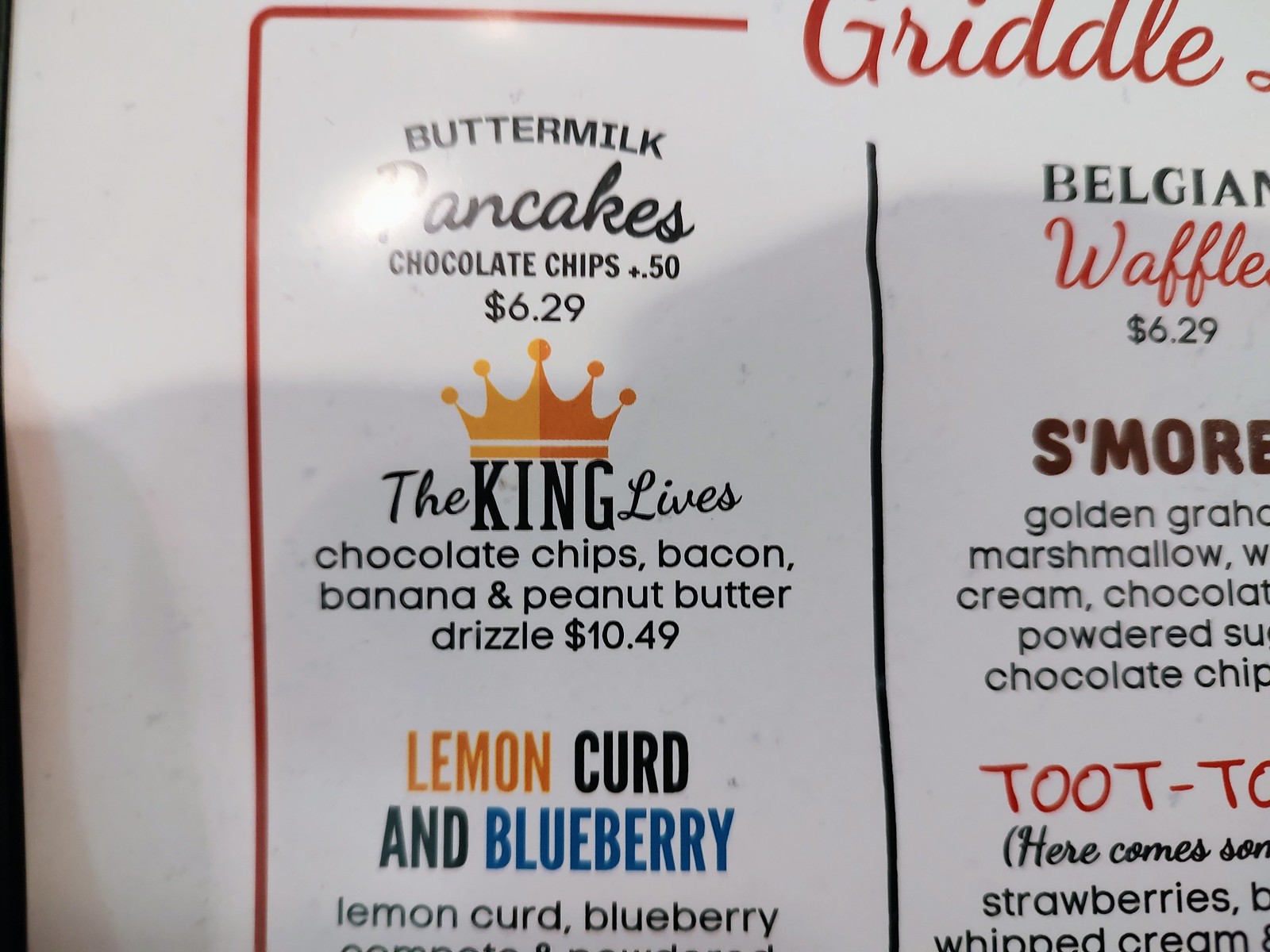This image showcases a restaurant menu board prominently featuring a variety of breakfast items, particularly different types of wheat-based foods. The sign itself is predominantly white and employs a mix of distinct fonts to highlight various sections and items. Central to the design is a square formed by two red lines—one vertical and one horizontal—alongside a black line. These lines converge near the word "Griddle," which is written in bold red, slightly off-center towards the middle of the image.

The left side of the menu board details several types of pancakes, referred to as "buttermilk pancakes," with customizable additions, including a special item called "The King." This section includes descriptive text in black beneath each food name, elaborating on the offerings. Additionally, there are partial glimpses of other menu items on the periphery, such as a "Belgian waffle," an item hinting at "s'more," and another intriguingly named "Toot" with a hyphen, although the full titles and descriptions are partially obscured.

Each item on the board is distinguished by unique fonts and colorings, making the menu visually engaging and easy to navigate for patrons.